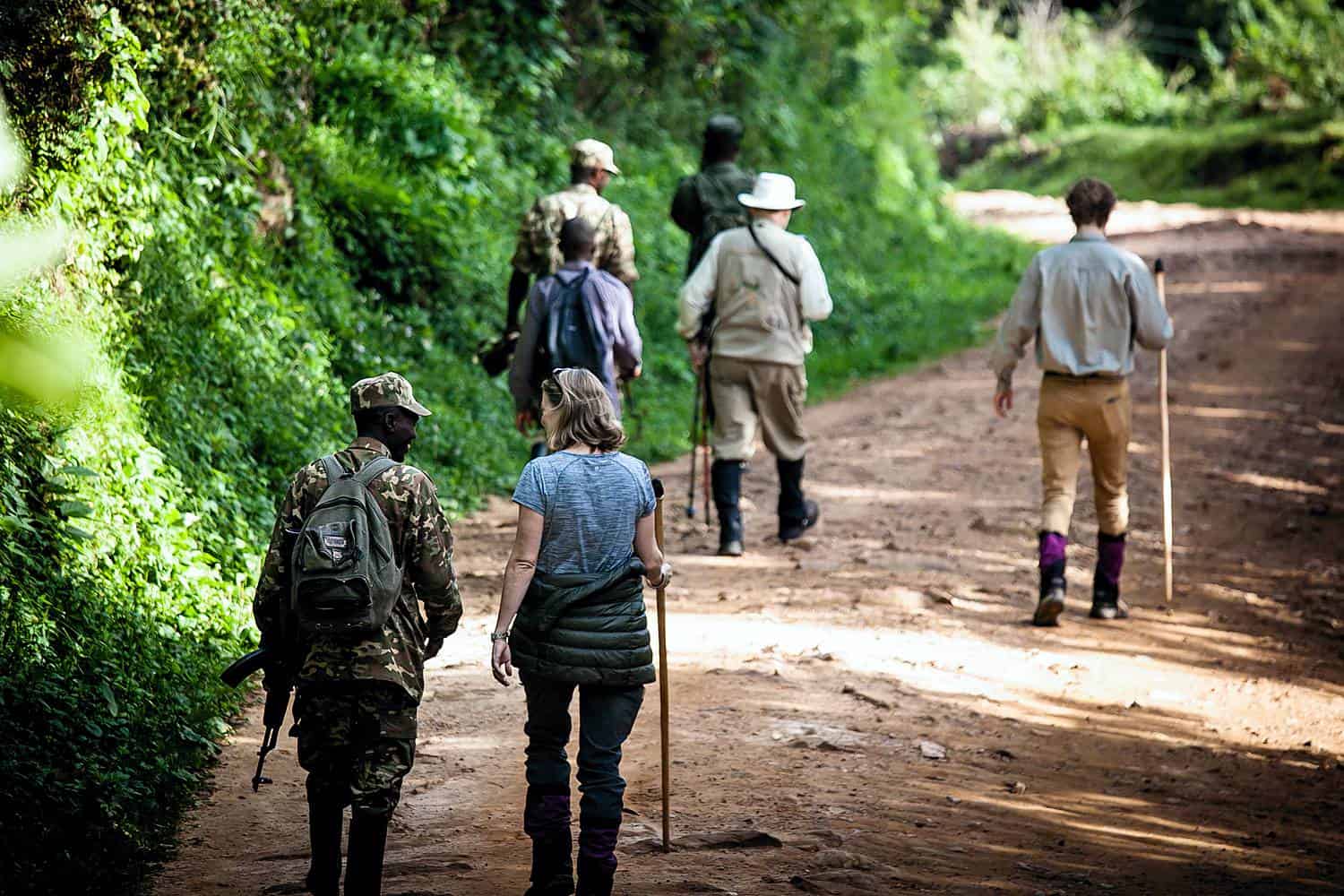A group of people, including what appears to be two military personnel and several civilians, are hiking along a rocky, curved dirt path flanked by lush green plants on the left. The two men in the front are wearing long black boots and carrying long stalks, while a man in camouflage gear, wearing a black backpack and seemingly armed, walks behind them. Next to him, a woman is talking to him and holding a long hiking stick. The scene appears to show a mix of locals and armed individuals, with the hikers looking somewhat tired as they move deeper into the forest. From the back, the assortment of hiking gear and the unexpected presence of armed men with backpacks lends a curious and somewhat uneasy atmosphere to the image.